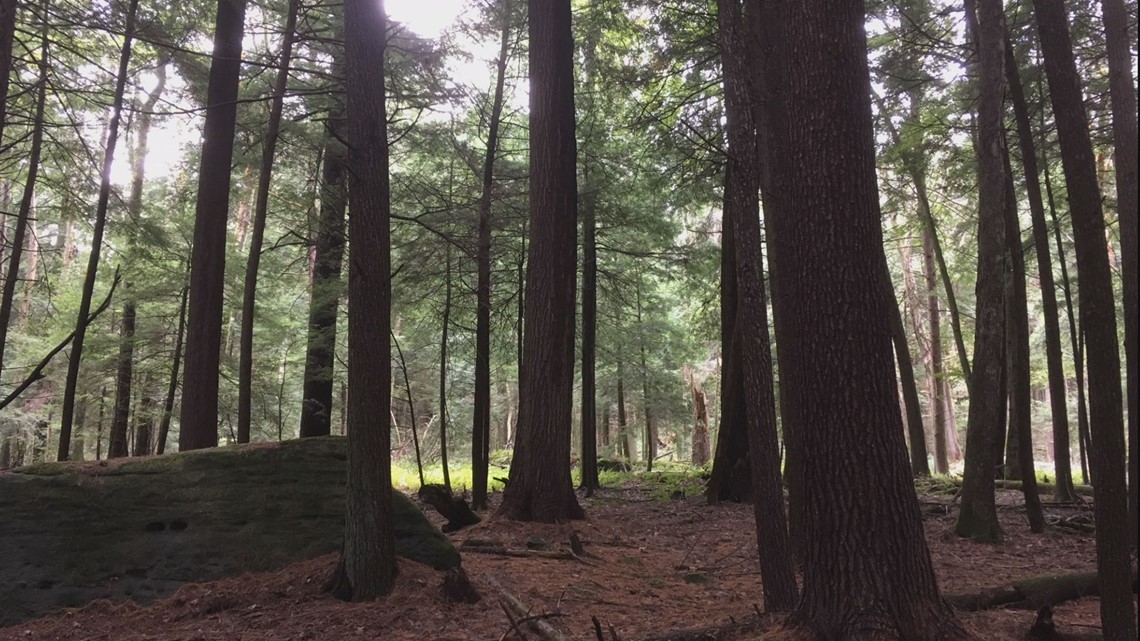This image captures a dense forest scene under a thick tree canopy, rendering the photo quite dark. The towering trees, mostly of thin to medium size with dark brown bark, are interspersed throughout the area, punctuated by patches of bright green grass visible in the distant background where sunlight penetrates the canopy. The sky is a bright white, peeking through the foliage, indicating it's likely morning. On the left side of the image, a fallen tree lies on its side, partially leaning against another tree, with additional logs and limbs scattered in the bottom corners of the frame. The ground is covered in a mix of dirt, branches, and pine needles, contributing to the forest's dark, lush atmosphere. The trees are adorned with green leaves, suggesting the season is spring or summer.